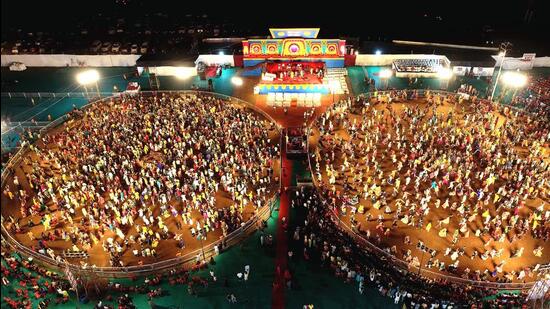The image captures an elevated, detailed view of what appears to be a large, festive event, potentially a concert or carnival, bustling with people. At the center of the scene are two large, circular enclosures filled with hundreds, perhaps even thousands, of attendees. Each circular area has a brown floor and is encircled by a curved barrier reminiscent of cattle pens.

Surrounding the circles and filling the gaps between them, a green floor stretches out, with a prominent red-colored walkway providing access through the middle. To the left, on the green surface, some tables are visible, while beyond the enclosures lies a red stage adorned with a blue trim at its base and colorful, Mexican-inspired flowery art on top. Atop the stage are bright lights, illuminating both the stage and the crowd below.

In the background, a parking lot dotted with cars is seen beyond a white wall, hinting at the venue's large capacity. The image, likely captured from a drone about 30 to 40 feet above ground, gives a comprehensive view of the entire lively area. People are not only inside the enclosures but also milling around outside, highlighting the event's vibrant and bustling atmosphere.